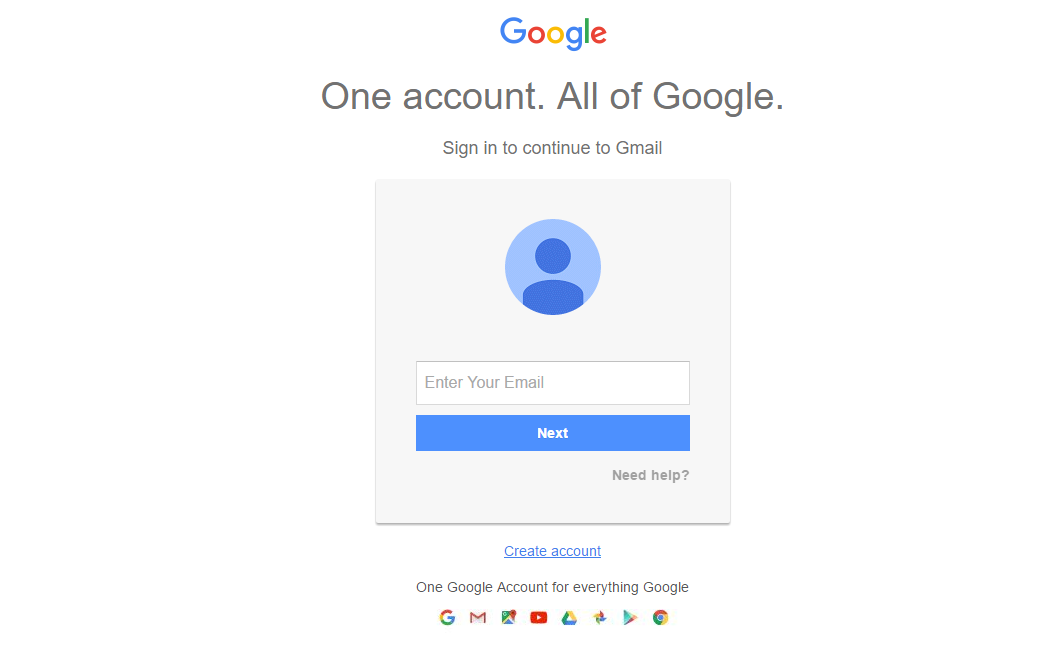The image depicts a Google sign-in page. The word "Google" is prominently displayed at the top, with the letters colored as follows: the first "G" is blue, the first "O" is red, the second "O" is yellow, the second "G" is blue, the "L" is green, and the final "E" is red. Beneath "Google," there's a statement in dark grey text that reads, "One account. All of Google."

In a smaller font below, there's a message, "Enter your email to continue to Google." This is followed by a grey box, within which sits a blue circle containing a smaller, darker blue circle, which symbolizes a person.

Below this graphic, there's a white rectangular input field with a grey outline, prompting users with the text "Enter Your Email." Below the input field, a blue button with white text says "Next."

To the right of the "Next" button, in grey text, is the phrase "Need help?" with a capital "N." Underneath this in blue, underlined text is the phrase "Create account" with a capital "C."

At the bottom, there's a black text statement declaring, "One account for everything Google," where each initial word is capitalized, and a list of Google services including Google Search, Gmail, Google Maps, YouTube, Google Drive, and Google Photos.